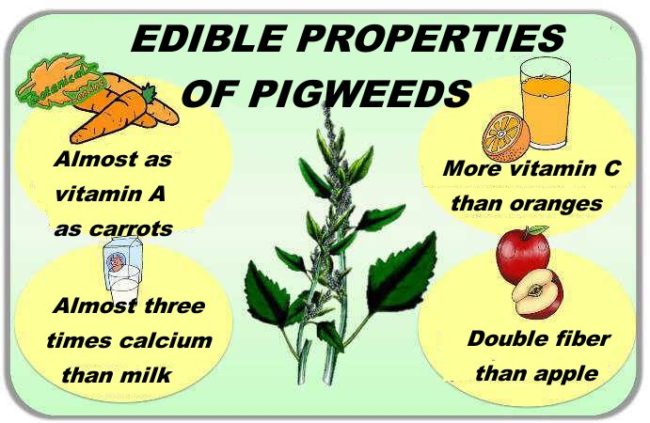The image, a cartoonish infographic, showcases the edible properties of pigweed. At the top, bold italicized black text reads "Edible Properties of Pigweeds" against a mint green background. In the center, a vibrant illustration of a pigweed is depicted with leafy green spade-shaped leaves and delicate purple flowers or berries. Surrounding the plant are four yellow ovals, each highlighting a specific nutritional benefit of pigweed.

- The top right oval features an image of half an orange and a glass of orange juice, with text stating "More vitamin C than oranges."
- The bottom right oval displays a whole red apple and an apple slice, accompanied by the text "Double fiber than an apple."
- The bottom left oval shows a carton and a glass of milk, with the text "Almost three times more calcium than milk."
- The top left oval depicts three orange carrots, stating "Almost as much vitamin A as carrots."

Despite minor grammatical errors in the original captions, the overall message emphasizes the impressive nutritional value of pigweed compared to common fruits and vegetables.